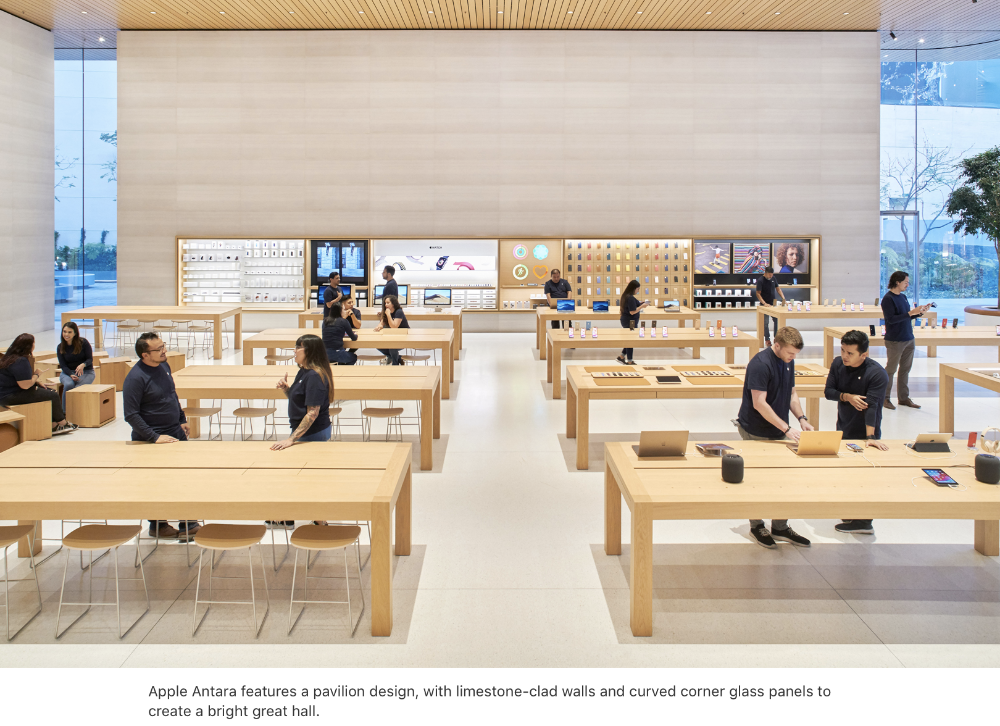This photograph captures a screenshot of a sizable building, specifically an Apple Store. The image showcases a group of people inside, highlighting the store's modern and inviting interior. The architectural design features a pavilion style with elegant limestone-clad walls and sleek, curved glass panels at the corners, creating a bright and spacious great hall. Abundant natural light streams into the space, illuminating the contemporary atmosphere. The store is furnished with wooden desks, adding to the warm and sophisticated ambiance. Overall, the rectangular-shaped photograph effectively conveys the store's impressive and welcoming environment.